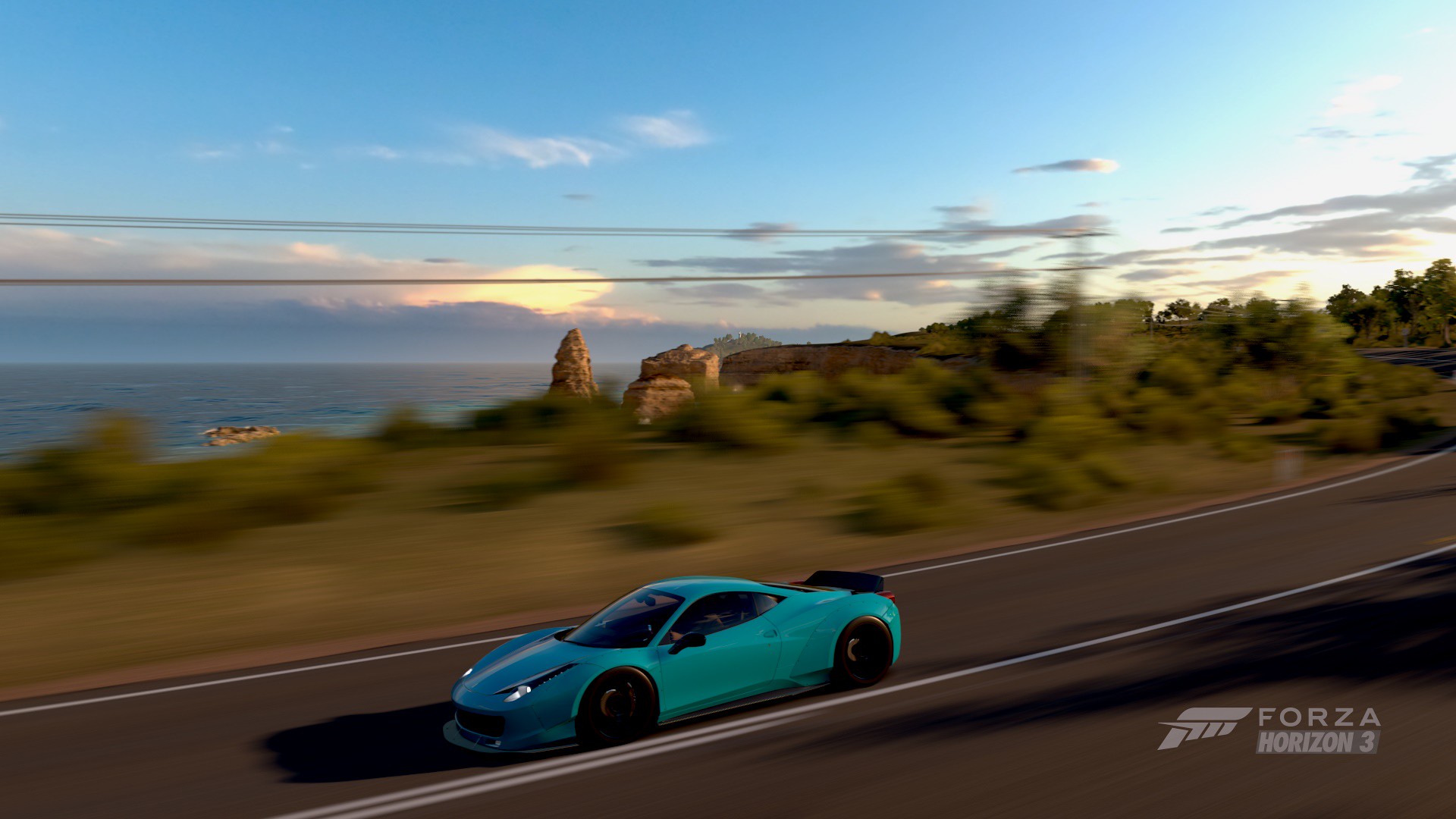In this detailed and vibrant screenshot from the video game Forza Horizon 3, a sleek aqua blue Ferrari 458 roars down a well-maintained, grey asphalt coastal highway. The car, a low-to-the-ground sports model, is accented with black tires and a matching black spoiler, giving it a sharp and aggressive look. The scene is set against a picturesque seaside backdrop, where a large body of water stretches out beneath a sky adorned with some grey-tinged clouds, hinting at a setting sun. The fast-moving vehicle leaves the background in a blur of green grass, shrubs, and rocky outcrops, suggesting a scenic route reminiscent of California's Highway 1 or perhaps a coastal road in Italy. The lower right corner of the image prominently displays the Forza Horizon 3 logo, confirming its origin in the acclaimed racing video game. The overall image captures the dynamic speed of the car and the stunning, realistic environment, highlighting the immersive experience of the game.